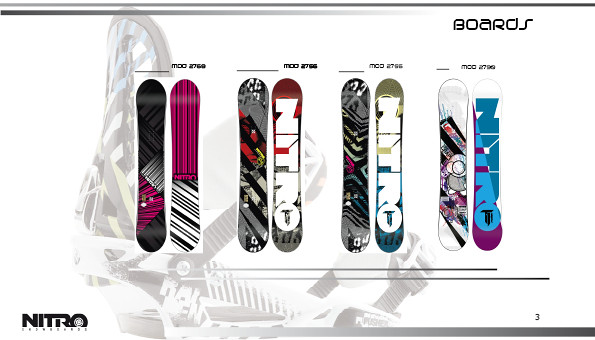In an eye-catching promotional image for Nitro snowboards, the advertisement displays four distinctive snowboard models, each shown from both the front and back. On the left, a pink and white snowboard with black accents stands out, labeled as Mod 2768. Beside it, the second board showcases a striking combination of red, gray, and black, identified as Mod 2766 in the center. Next is the green and blue Mod 2766, and finally, a vibrant design featuring blue, purple, white, and some red and gray, known as Mod 2790. All boards prominently display the Nitro branding, with the brand name visible on each board. The background is adorned with a subtle, gray graphic, adding depth to the display, while the words "boards" are seen at the upper right corner of the ad. In the bottom left corner, the NITRO logo is prominently positioned in black, encapsulating the brand's identity.